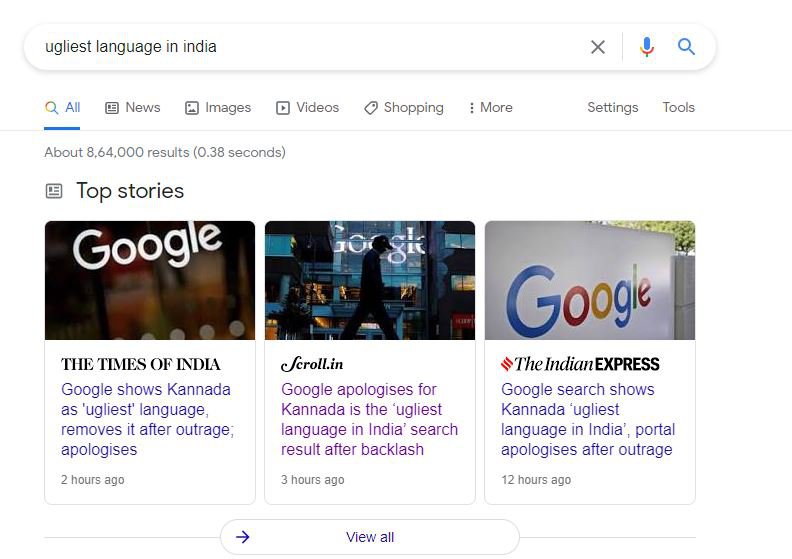A screenshot shows Google search results for the query "ugliest language in India." The results appear immediately after the search was made, with a reported 864,000 results found in just 0.3 seconds. The page displays a list of top stories, including three thumbnail images with the Google logo, each linked to a news article.

The first thumbnail, showing the Google logo against a broken background, is from The Times of India, with the headline, "India shows Kannada the ugliest language and moves it after outrage, apologizes," published two hours ago. The second image from Scroll.in depicts a man walking in front of a Google building with the logo visible through a glass wall, accompanying the headline, "Google apologizes for Kannada is the ugliest language in India. Search results after backlash," posted three hours ago. The third image from The Indian Express shows a Google sign outside, adjacent to a cemented area, with the accompanying headline, "Google shirts shows Kannada ugliest language in India. Google apologizes after outrage," published 12 hours ago.

Below these top stories is an option to "View All," indicated by an arrow pointing to the right.